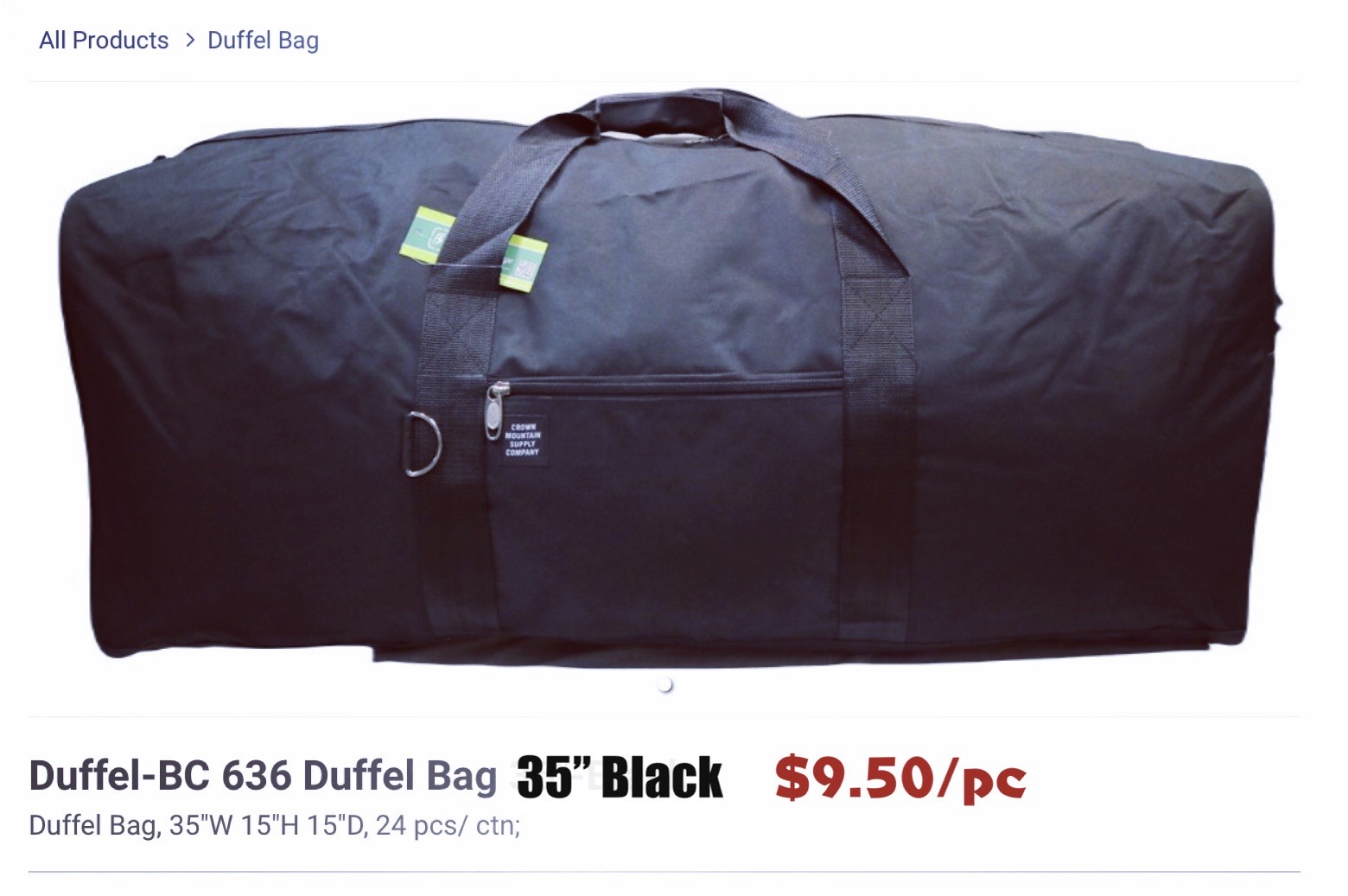This close-up, color photograph serves as an advertisement for a dark blue duffel bag, prominently featuring its details. The main duffel bag is rectangular and navy blue with a short dark blue strap that functions as the handle. It also has a side pocket with a silver horizontal zipper. The small rectangle tag on the bag reads "Crown Mountain Supply Company" in white text. A rectangular patch in blue and green is tucked behind the handles, partially obscured by the strap. The caption details the product as "Duffel BC636 Duffel Bag, 35 inches black," priced at $9.50 per piece. The dimensions of the bag are provided, measuring 35 inches wide, 15 inches high, and 15 inches deep, with 24 pieces included per carton. At the top of the advertisement, the navigation path on the website says "All Products" followed by an arrow leading to "Duffel Bag."